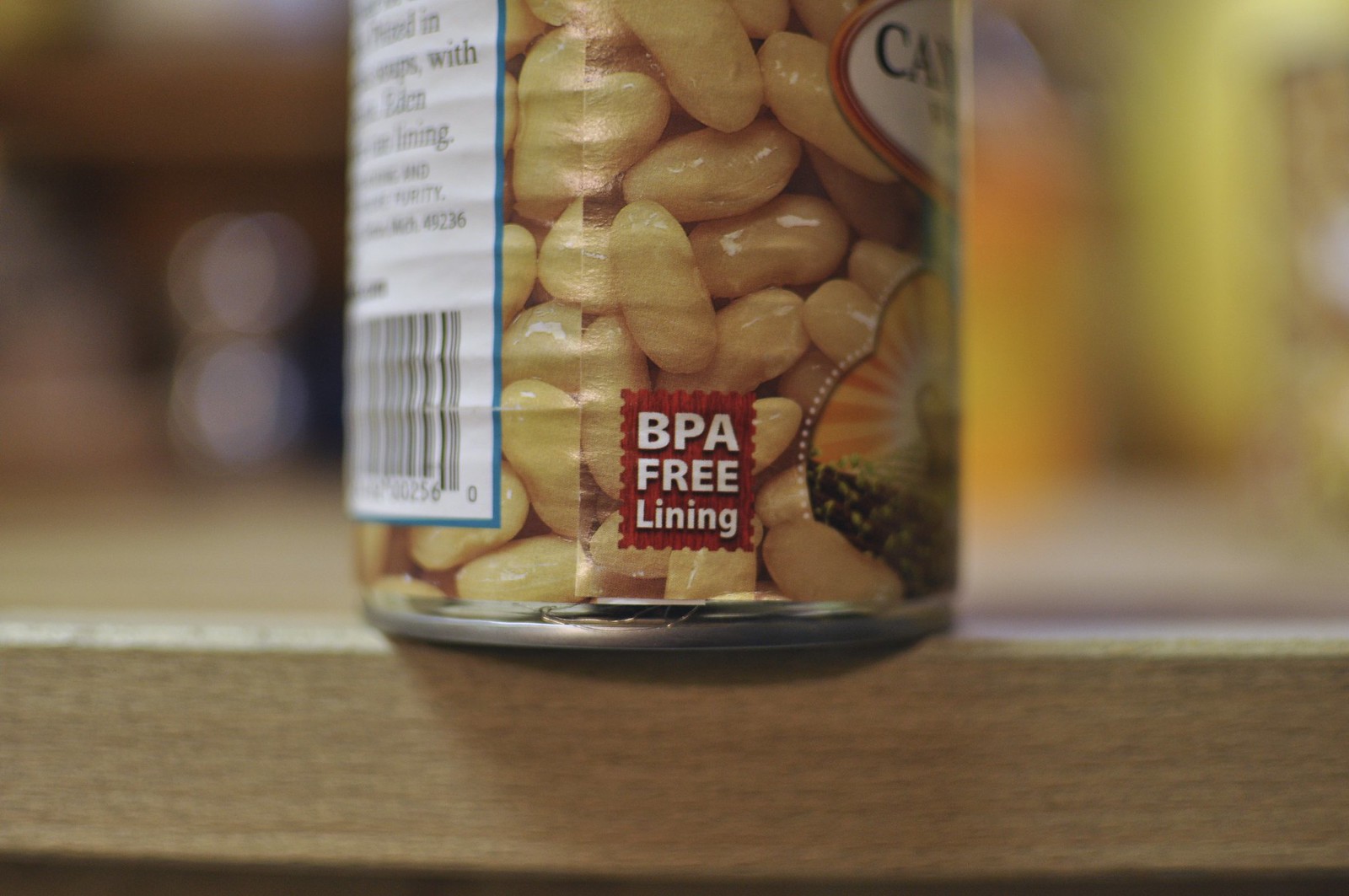The image features a detailed close-up of a can of white beans, likely either cannellini or great northern beans, with a distinct tan and yellow hue possibly influenced by the lighting. The can is positioned at a three-quarter angle, revealing several key details of its label and packaging. A prominent part of the label includes a small, stamp-shaped red square with white text reading "BPA-free lining," emphasizing the can’s safe packaging. On the lower left, a partially visible barcode appears, while to the right, there is a glimpse of the nutrition information in a large white rectangle bordered in blue.

The central background of the can’s label is a vivid image of the beans themselves. Toward the top right, partially visible, is the brand or product designation starting with "CA" in dark green lettering. Adjacent to this is an illustrated logo depicting a stylized farm scene with a setting or rising sun, emitting red and yellow rays, encapsulated in a cloud-like shape with a striped pattern of alternating orange and burnt orange stripes. Below the branding, a subtle but noticeable dark green and light green foliage design can be observed. The can rests on a light wooden desk, with the background blurred to keep the focus on the intricate label details.